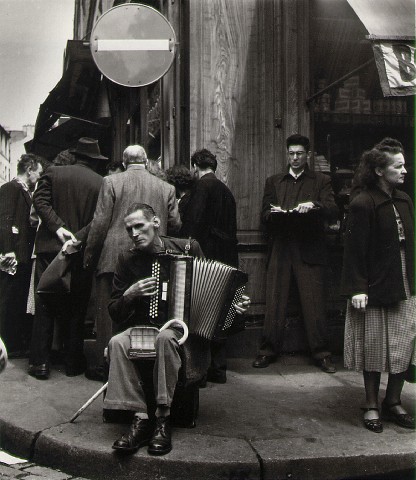This black-and-white photograph, likely taken in the 1940s based on the attire, captures a bustling urban scene centered around a man playing an accordion while seated on a concrete sidewalk. He wears a dark shirt, light pants, and black shoes. Directly to his left stands a woman in a black coat over a white or gray dress, looking away from him. Behind her is a man in a jacket and gray slacks, holding a book or paper. A group of men are gathered behind and to the left of the accordionist, engrossed in something on the ground, possibly a card game or another street performance, their backs turned to the camera. Above this gathering, a circular European-style stop sign with a line through it is visible. The backdrop of the scene includes a storefront with a partially visible sign starting with the letter "B" and features wooden drawers and cupboards, hinting at a bookstore or similar establishment. The crowded street exudes a lively atmosphere, typical of people engaging in various urban activities.